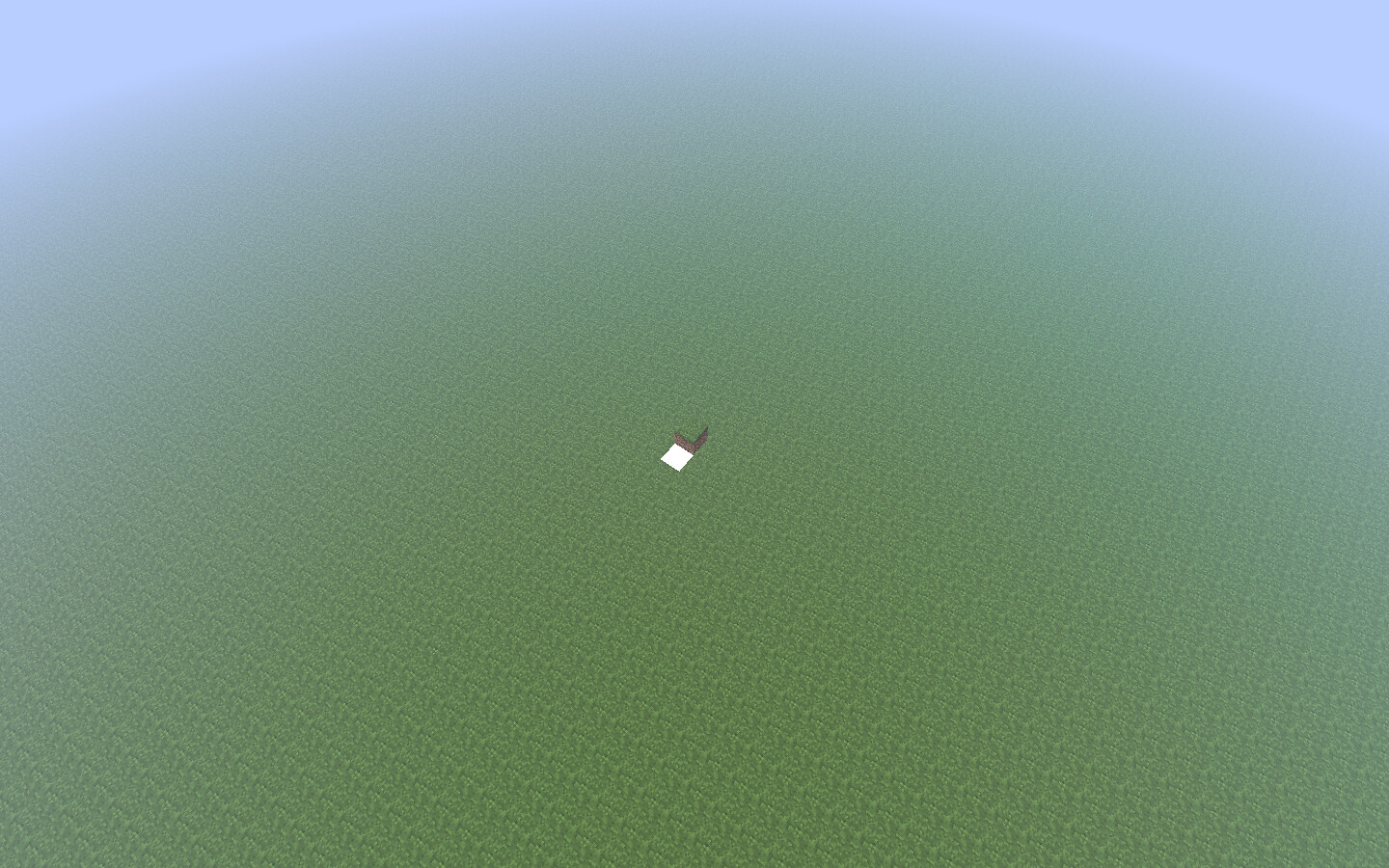A rectangular image with its long axis positioned horizontally dominates the frame. The scene is predominantly green, featuring a subtly textured surface that gradually transitions into a solid sky blue near the top, especially in the top two corners. At the center, a white square is accompanied by a cube-shaped object exhibiting a green top and brown sides, characteristic of a grass block from the game Minecraft. There is no visible user interface, suggesting that this is a clean screenshot from Minecraft, highlighting a simple yet familiar element from the game.